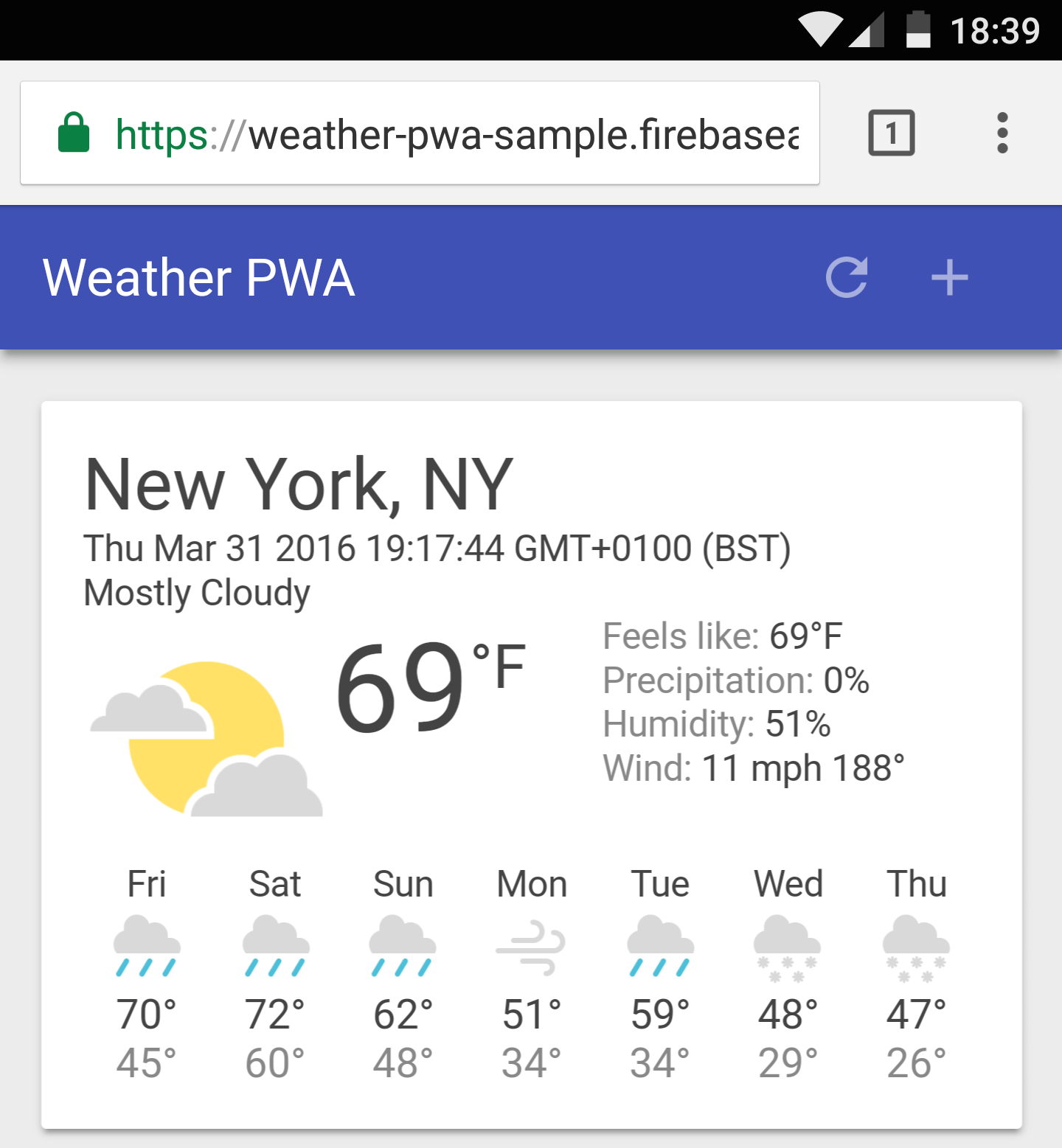**Descriptive Caption:**

This image is a screenshot of a user's phone displaying a web browser currently navigated to a partially visible URL, "weatherpwasample.firebase...". The browser's top left corner includes a blue header with white text reading "weatherpwa," accompanied by a refresh icon and an ad icon. Below the header, the weather forecast for New York, New York is presented. The date is Thursday, March 31, 2016, and the time is 19:17 GMT.

The current weather is mostly cloudy with a temperature of 69°F, which also feels like 69°F. Additional weather details include 0% precipitation, 51% humidity, and wind blowing at 11 mph from 188 degrees. The upcoming forecast indicates:

- **Friday:** Rainy, 70°F
- **Saturday:** Rainy, 72°F
- **Sunday:** Rainy, 62°F
- **Monday:** Windy, 51°F
- **Tuesday:** Rainy, 59°F
- **Wednesday:** Mixed snow flurries, high of 48°F and low of 29°F
- **Thursday:** Similar snowy conditions, high of 47°F and low of 26°F